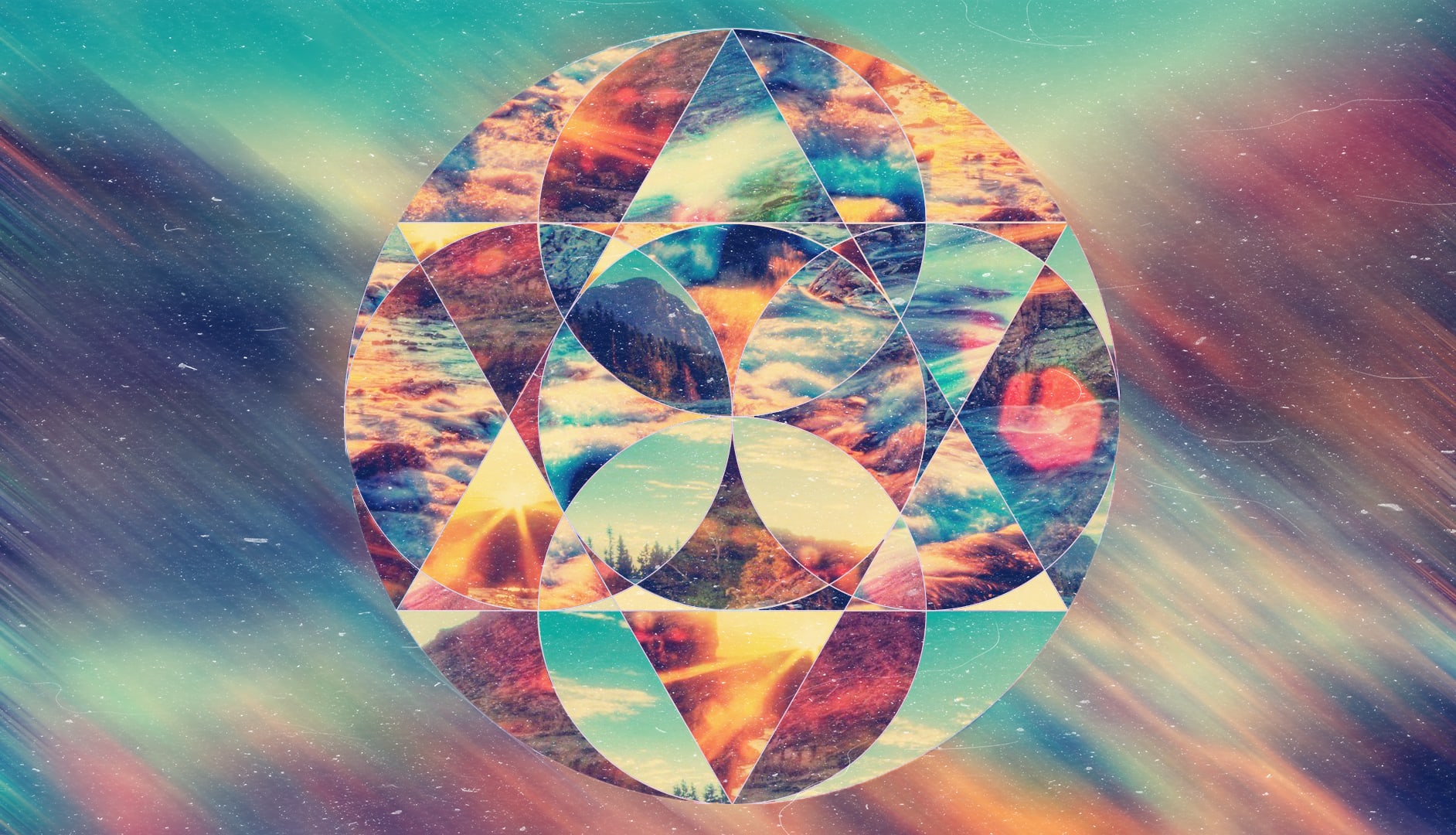This image features a large circle composed of various geometric shapes, primarily rectangles and triangles, all intricately arranged in a dynamic, collage-like pattern. The circle showcases a vibrant spectrum of colors, including blue, orange, yellow, red, and teal, with teal prominently positioned towards the top. The overall composition is highly artistic, blending multiple shapes and hues into a cohesive, visually stimulating whole. The backdrop is a rich maroon color, which contrasts sharply against the colorful, geometric focal point, enhancing the image's depth and complexity.